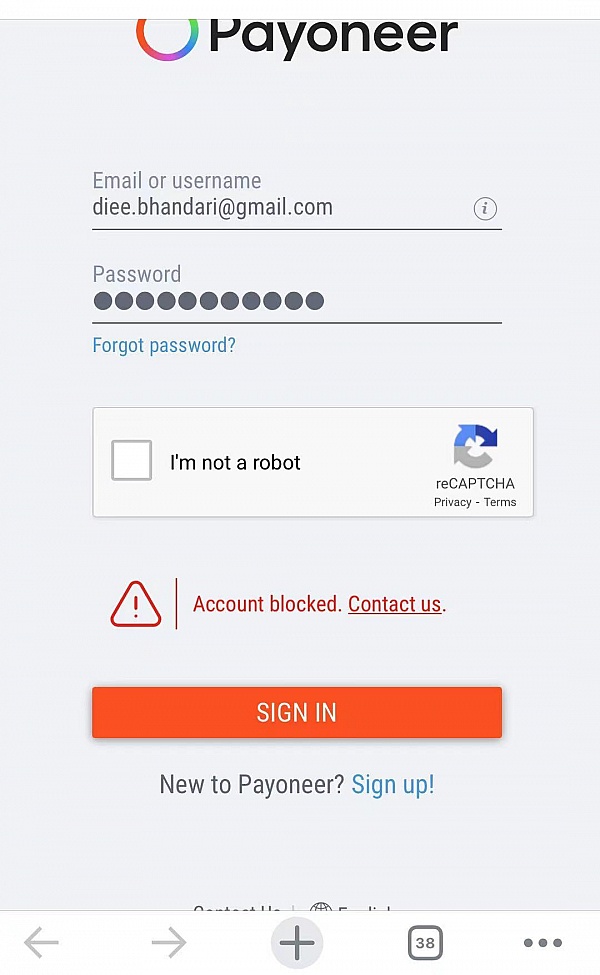The web page for the product Payoneer features a partially visible circle logo on the top left, showcasing colors of orange, blue, and green. To its right, the word "Payoneer" appears in black lettering, with the top part of the letter "P" cut off. Below the logo, there is a sign-in form with a light blue background.

The sign-in section includes:
1. A field labeled "Email or Username" with a sample email entered.
2. A field labeled "Password" with around 10-11 gray circles indicating the password input.

Beneath the password field, there is a gray horizontal line spanning the width of the form. Below this line, a blue link labeled "Forgot Password?" is apparent.

Further down, the page presents a reCAPTCHA section with a checkbox labeled "I'm not a robot" accompanied by two blue arrows pointing to the right, indicating verification. There is a statement "reCAPTCHA privacy terms" nearby.

Below the reCAPTCHA, there is a highlighted warning section on the left with a red triangle icon containing a question mark and a red alert message: "Account blocked Contact us".

At the bottom of the form, an orange banner displays a white "Sign In" label. Beneath the banner, there is a prompt in gray/blue text stating "New to Payoneer?" followed by a blue "Sign Up!" link.